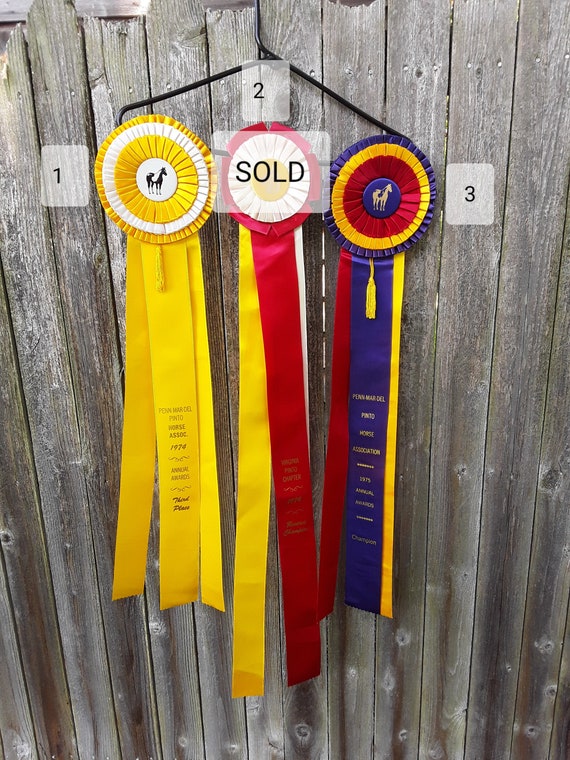The close-up photograph showcases a worn, grey-brown wooden fence made of narrow vertical planks, each with visible knots towards the bottom. Two nails are side-by-side at the top of one plank. Hanging from the fence on a wire rack are three colorful ribbons indicating awards. They are spaced slightly apart, fanning out for display, and each ribbon bears a number and text. The left ribbon is gold-yellow and displays the text "Penn-Mar-Cal-Pinto-Voors Association, 1974," indicating it might be from a past event, likely a 4-H or Pinto Horse Association annual awards. The middle ribbon, predominantly red with some yellow and white, has "sold" written in black text and bears the number 2. The rightmost ribbon features blue, yellow, and red colors with a hint of gold and is marked with the number 3. The overall scene suggests an outdoor setting, possibly resembling a yard sale or flea market, and focuses solely on these three award ribbons hanging on the fence.